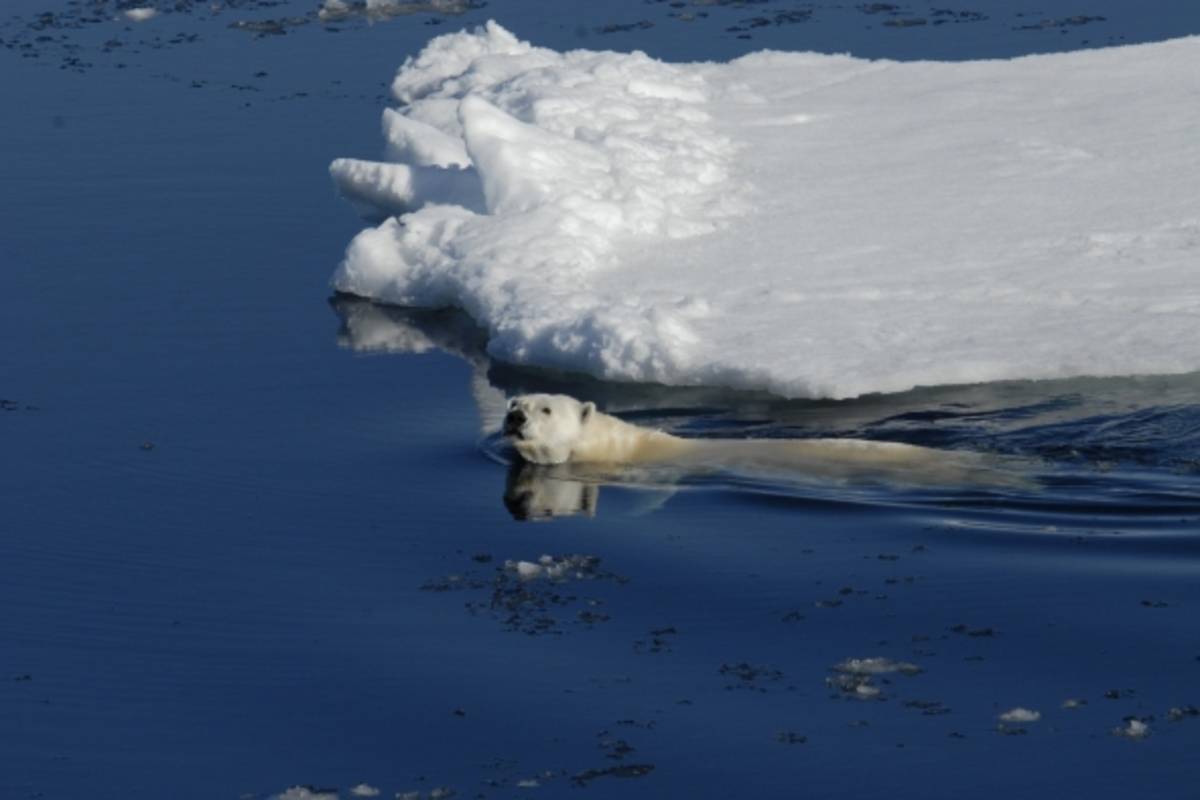In the bright, sunny daytime, a large polar bear swims in the deep, dark blue ocean waters, surrounded by sparse, tiny chunks of ice. Most of the polar bear's body is submerged, with primarily its head and a bit of its back visible, including its black nose and dark eyes. Reflected in the water, the bear seems to be swimming toward the left of the image. On the right side of the picture, there is a large, flat chunk of ice that doesn't extend across the entire screen, leaving the left side predominantly filled with water. Along the top portion of the image, there's a distant strip of water visible beyond the ice, emphasizing the isolated and vast nature of the scene.